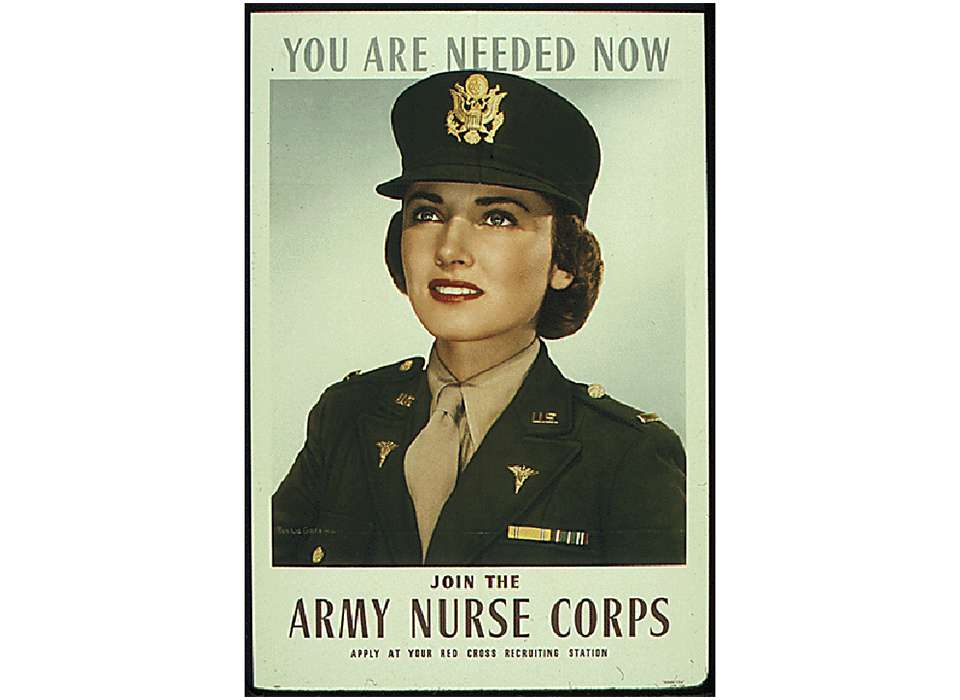The image is a vintage or reproduction poster advertising for the Army Nurse Corps. The background is a pistachio green, bordered at the top by a darker sage green banner that reads "You are needed now" in capital letters. The poster features a central figure of a woman dressed in a tan uniform, including a tan-colored top with a matching tie. She wears a black hat adorned with a gold emblem reminiscent of a government eagle, and a matching tan suit jacket decorated with various medals on both sides. The woman has red lipstick and short, cropped hair, and additional emblems on her shoulders and collar. At the bottom of the image, a banner reads "JOIN THE ARMY NURSE CORPS" in capital letters, followed by "Apply at your Red Cross recruiting station." The entire poster is enclosed in a thin black frame.